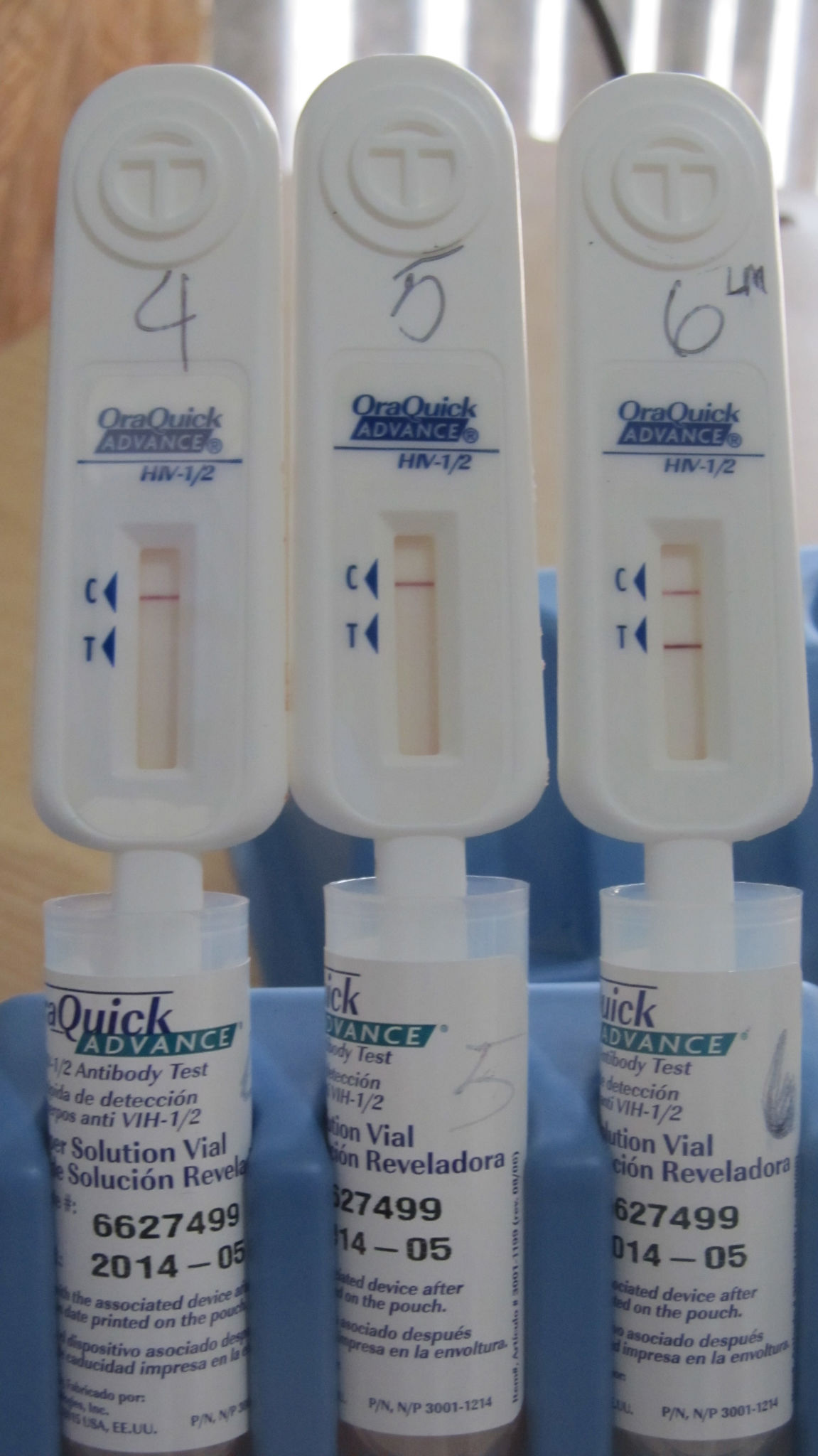The image showcases three Quick-Advance rapid antibody tests, specifically labeled as "Quora Quick-Advance HIV 1/2." These tests, which resemble pregnancy tests, are numbered 4, 5, and 6 and are standing upright in individual vials. In the test window area, each has markings labeled "C" (Control) and "T" (Test) with arrows pointing to them. All three tests have a line next to the "C," indicating the control test has worked correctly. Notably, test number 6 also has a line next to the "T," suggesting a positive indication for HIV antibodies. The tests are held in place by a blue holder, and the setting appears to be indoors with wooden accents and blinds evident in the background, illuminated by natural light. The tests are neatly arranged in numerical order from left to right.